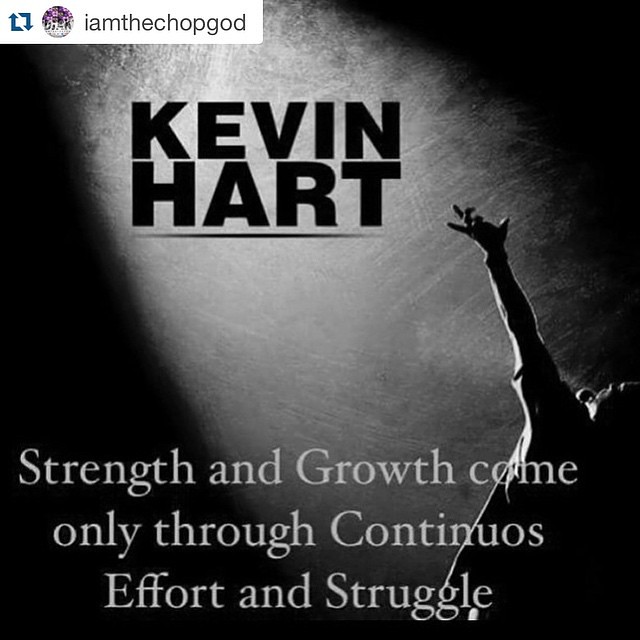The black-and-white image appears to be a promotional photo featuring comedian Kevin Hart. Dominated by shadows, the image shows Kevin Hart with his back and side facing the camera, his left arm outstretched towards a spotlight that dramatically highlights him. In his right hand, close to his mouth, he holds a microphone. Below this striking visual, a motivational quote in white text reads, "Strength and growth come only through continuous effort and struggle," though 'continuous' is misspelled as 'contiuous'. The text is irregularly capitalized, enhancing the quote's visual impact. In the top left corner, a colorful circular icon of uncertain detail is paired with a reshare symbol and the text "I am the Chop God," suggesting that the image was created and circulated by an entity or person known as the Chop God.